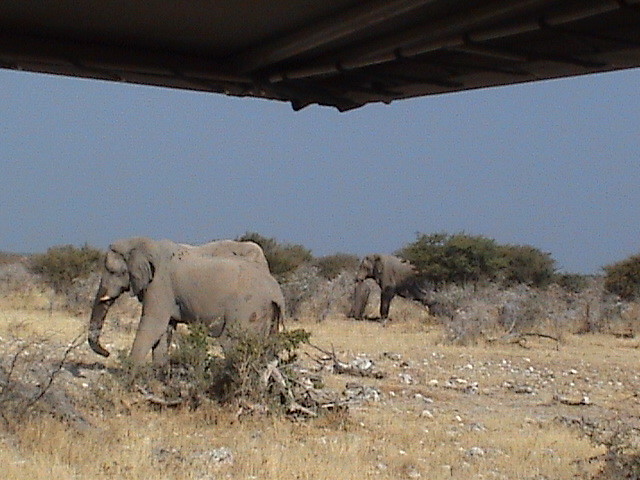In this detailed outdoor image, set against a clear, cloudless blue sky, we see two gray elephants on an African savannah. The background consists of lush, green trees interspersed with tall, brown, and gray dried weeds, sticks, and dirt. The foreground features a pile of broken logs and twigs, where one elephant, with a noticeable lump on its back, stands. The elephants are positioned as if viewed from under a rooftop or canopy, possibly of a Jeep. The elephant closer to the left has a trunk that appears brown, likely due to being wet, and it also has small white tusks. Both elephants are facing left and walking straight across the dry, shrub-filled area, which includes stones or possibly bones scattered around. The scene captures a serene moment of these majestic creatures in their natural habitat.